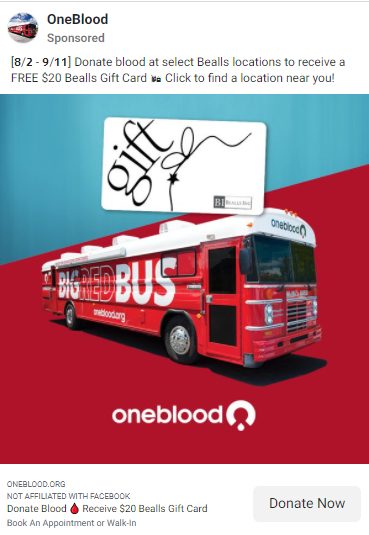This image is a digital advertisement for OneBlood, highlighting a blood donation campaign running from August 2nd to September 11th. The ad prominently features a photograph of a large red bus, known as the "Big Red Bus," with "OneBlood Sponsored" written at the top of the image. The background is divided into blue and red sections, with the OneBlood logo visible. Above the bus, there is an illustration of a gift card. The text informs viewers that donating blood at select Beals locations will earn them a free $20 Beals gift card and invites them to click to find a nearby location. Additional text at the bottom of the ad reads "OneBlood.org, not affiliated with Facebook," and includes a call to action to "Donate Now," likely referring to both blood and potential cash donations.